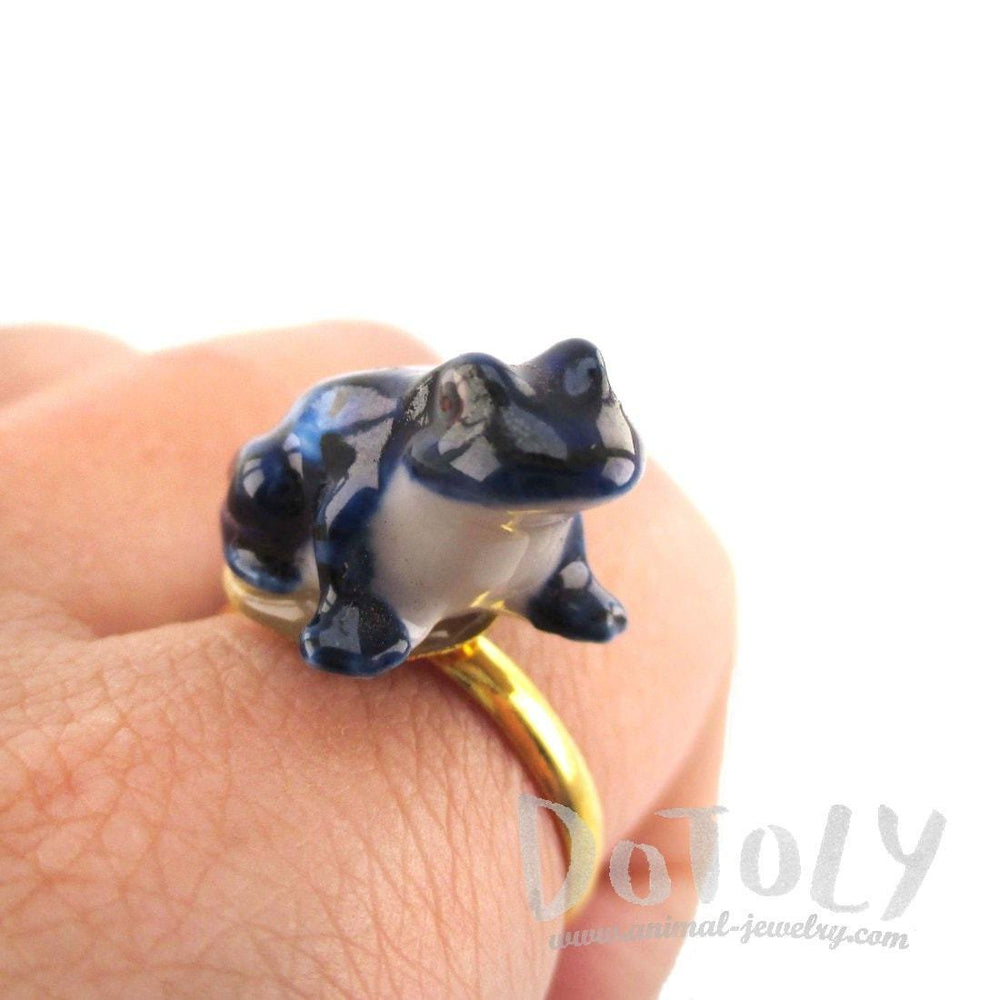The advertisement features a detailed close-up of a striking gold ring adorned with an intricate, glass-like frog design. The frog, which appears to be made of shiny glass, showcases a vivid blue body with a contrasting white underbelly. It possesses four legs and prominent red eyes that stand out against its glistening surface. The ring is modeled on a person's hand, which is depicted with fingers bent over the palm, showcasing the ring prominently at the center of the image. The background is a clean, stark white, providing a clear view of the jewelry. In the lower right corner, subtle silver-gray text reads "Dotali" with the website "www.animal-jewelry.com" slightly beneath it, nestled discreetly against the white backdrop.